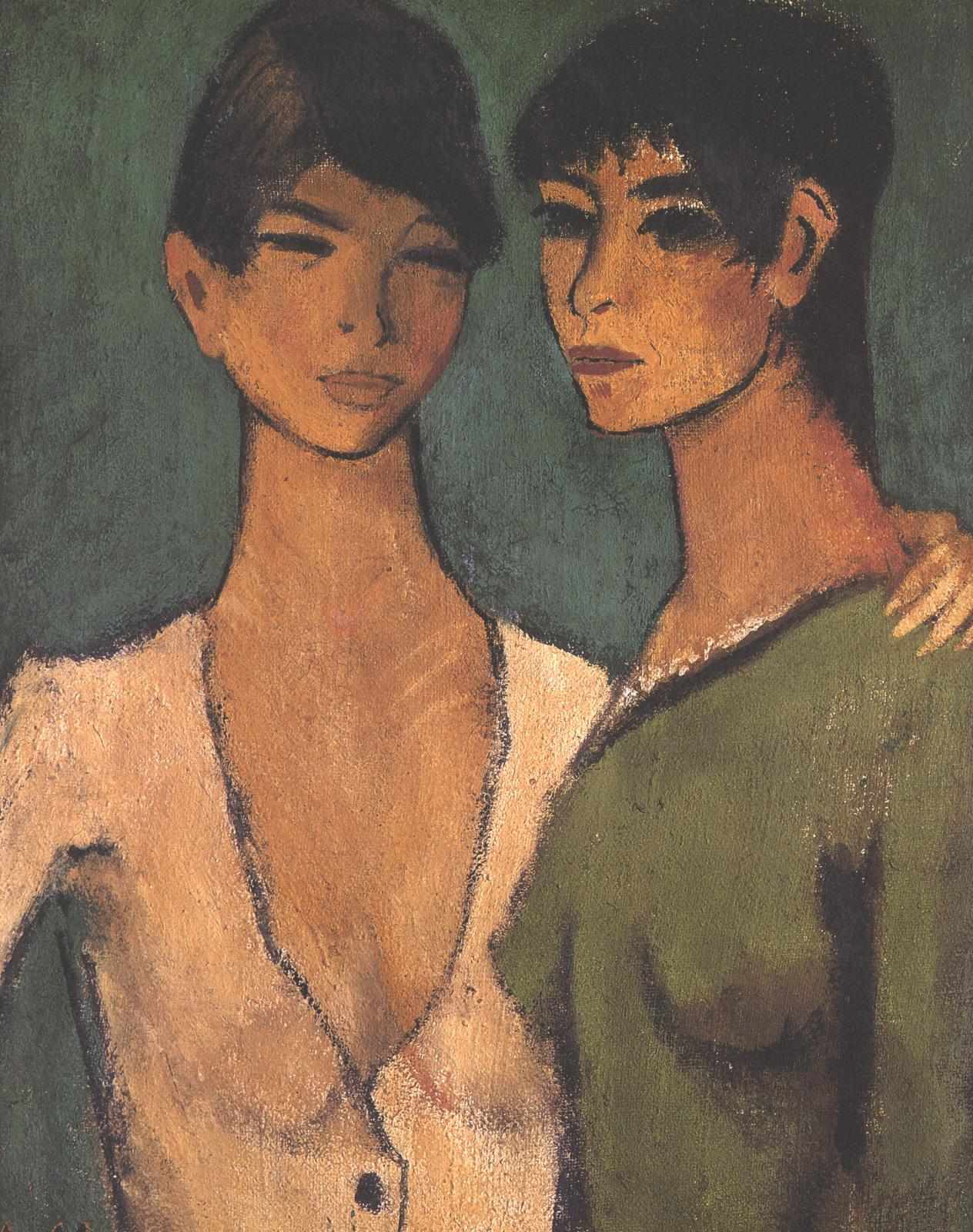The image is a drawing with a greenish-gray background, featuring two women in a cubist style, reminiscent of early 20th-century art. The woman on the left, characterized by her short brown hair, has closed eyes and a serene expression. She is wearing a beige cardigan with a V-shaped collar and buttons up, and she has her left arm placed tenderly on the shoulder of the woman on the right. This right-hand woman has long black hair that reaches down to her legs and is gazing thoughtfully towards the left of the image. She is dressed in a dark green top, and her expression remains neutral as she stands close to the other woman. The overall composition is abstract with limited detailing, emphasizing the intimate, yet contemplative connection between the two figures.